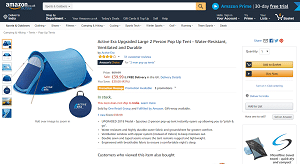A small image taken from the Amazon website depicts a product page featuring a two-person tent. The tent, varying in shades of blue—dark navy, royal, and sky blue—stands out against the typical Amazon page layout. On the left side of the image, a series of thumbnails are visible, presumably showing different angles and features of the tent. At the top of the main image, the product's rating is displayed, hovering around four out of five stars. Below the rating, the price is listed, accompanied by a promotional discount indicated in red text. The product is confirmed to be in stock, although the exact description remains unreadable due to the image's small size.

To the right of the main product image, orange "Add to Cart" and "Buy Now" buttons are prominently displayed, with possible social media sharing icons positioned above them. An advertisement occupies the bottom right corner, but its content is indistinguishable. 

The top right corner shows the user is currently enjoying a free trial of Amazon Prime, with the remaining days of the trial mentioned. The Amazon Prime text is in blue and is located to the right of the main Amazon search box. The shopping cart icon below indicates there are four items in the user's cart, as shown by the number above the cart icon.